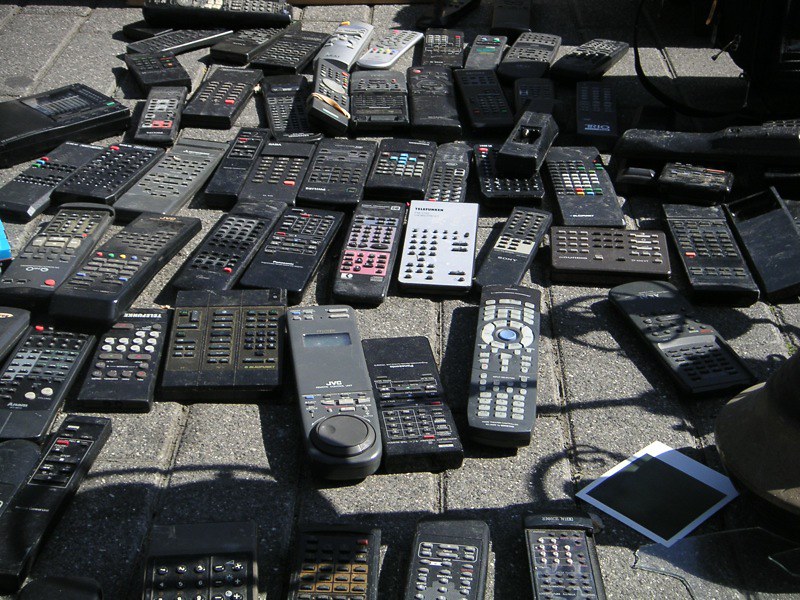The image features an extensive array of old-style calculators, remote controls, and possibly a few adding machines, all spread out on a gray, stone or concrete brick surface, likely in a courtyard or similar outdoor space. The devices, mostly black with a few silver or gray ones mixed in, display various designs, from rectangular shapes to those with round buttons at the bottom. Many of the devices are dusty and dingy, emphasizing their age. They are arranged in roughly six rows, with approximately 10 items per row, totaling around 40 to 50 pieces. The bright sunlight illuminates most of the scene, casting a few shadows here and there. Notably, a Polaroid photo, seemingly undeveloped, lies in the lower right corner, adding to the eclectic mix of objects. The buttons on the remotes and calculators are predominantly white or black with white lettering, and some feature a few red buttons. Overall, it appears that these items might be laid out for a sale or display.